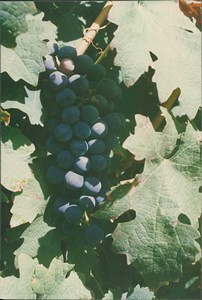This is a small, faded photograph of a grapevine on a sunny day. At the center of the image, there is a bunch of approximately 30 plump, ripe, and slightly dusty purple grapes, with one grape appearing a redder hue. The grapes are surrounded by large, light green leaves, which can be identified more by their texture than their color due to the faded quality of the image. The sunlight filters through the leaves, casting shadows on some of the grapes and giving the scene a yellowish tint. The brown stems and a bit of the vine are visible, mostly around the perimeter of the photo. Overall, this image captures a serene moment in a grape orchard, with the central focus on the ripening grapes nestled among lush foliage.